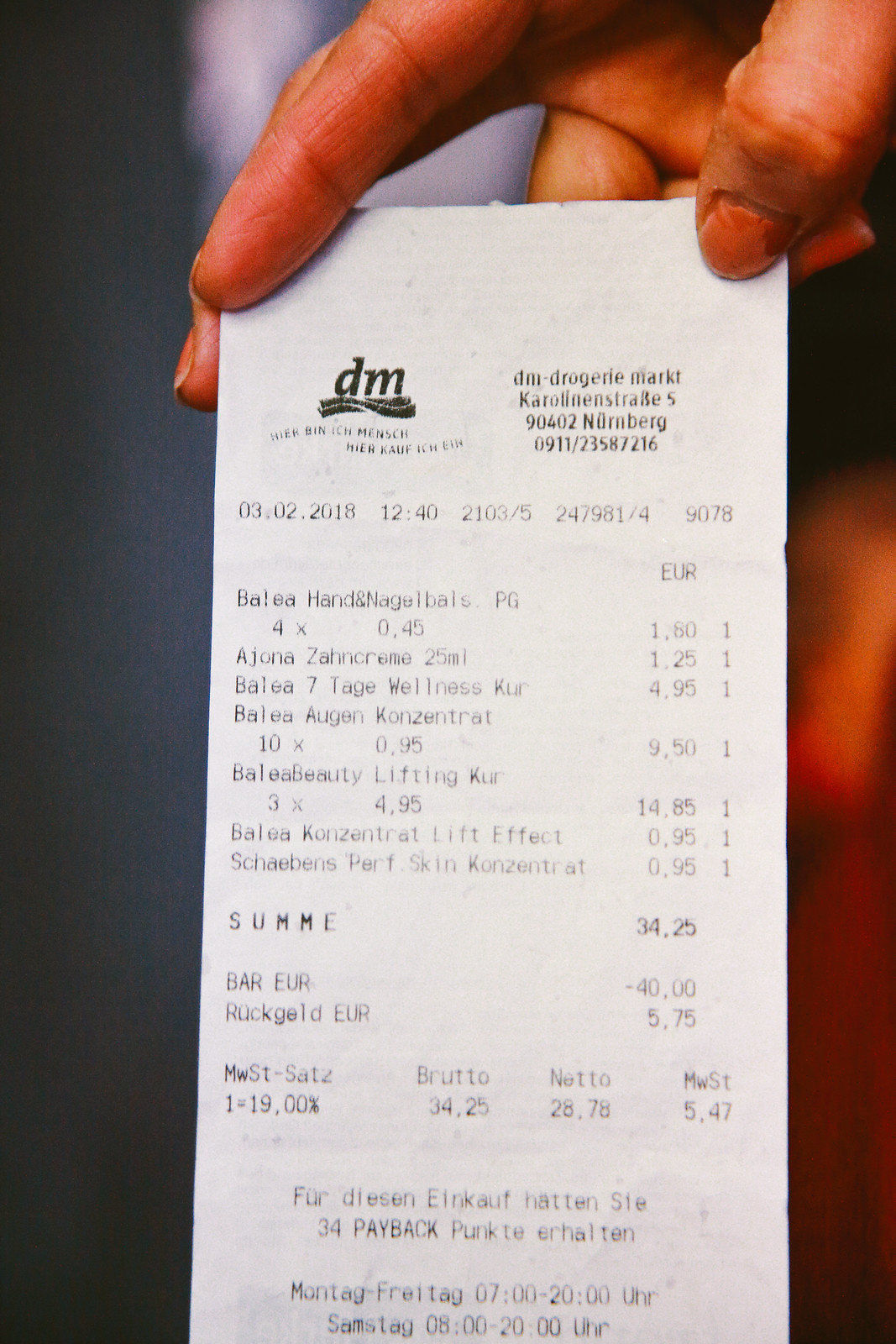The image showcases a crisp white receipt printed in black ink, being held by a woman's hand. Her nails are painted a vibrant pinky-coral shade. She grips the receipt delicately between her thumb and the first two fingers. At the top of the receipt, there is bold black lettering featuring the characters "D" and "M" with a small banner below, likely indicating the name of the establishment, which appears to be German. The receipt details several itemized purchases, each listed alongside their respective prices in Euros. Towards the bottom, additional text in German is visible.